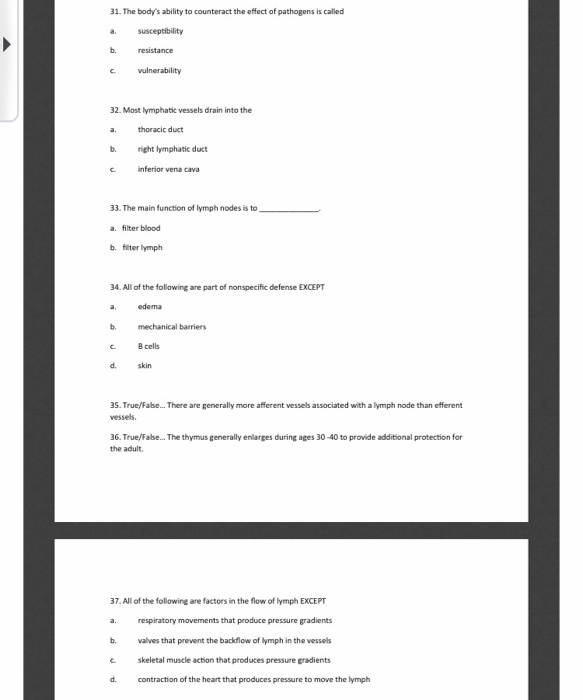The image features a grid-like layout segmented by grey bars on the sides. In the top left corner, there is a solitary black arrow. The rows are numbered from 31 to 37. Each row appears to correspond to a question, with multiple-choice options presented in columns. Specifically:

- Questions 31 and 32 offer choices labeled A, B, and C.
- Question 33 provides options A and B.
- Questions 34 and 37 have four choices each: A, B, C, and D.
- Questions 35 and 36 seem to be true-false questions, as indicated by the visible labels "True" and "False."

The textual content is predominantly in black, although much of it is challenging to discern clearly.